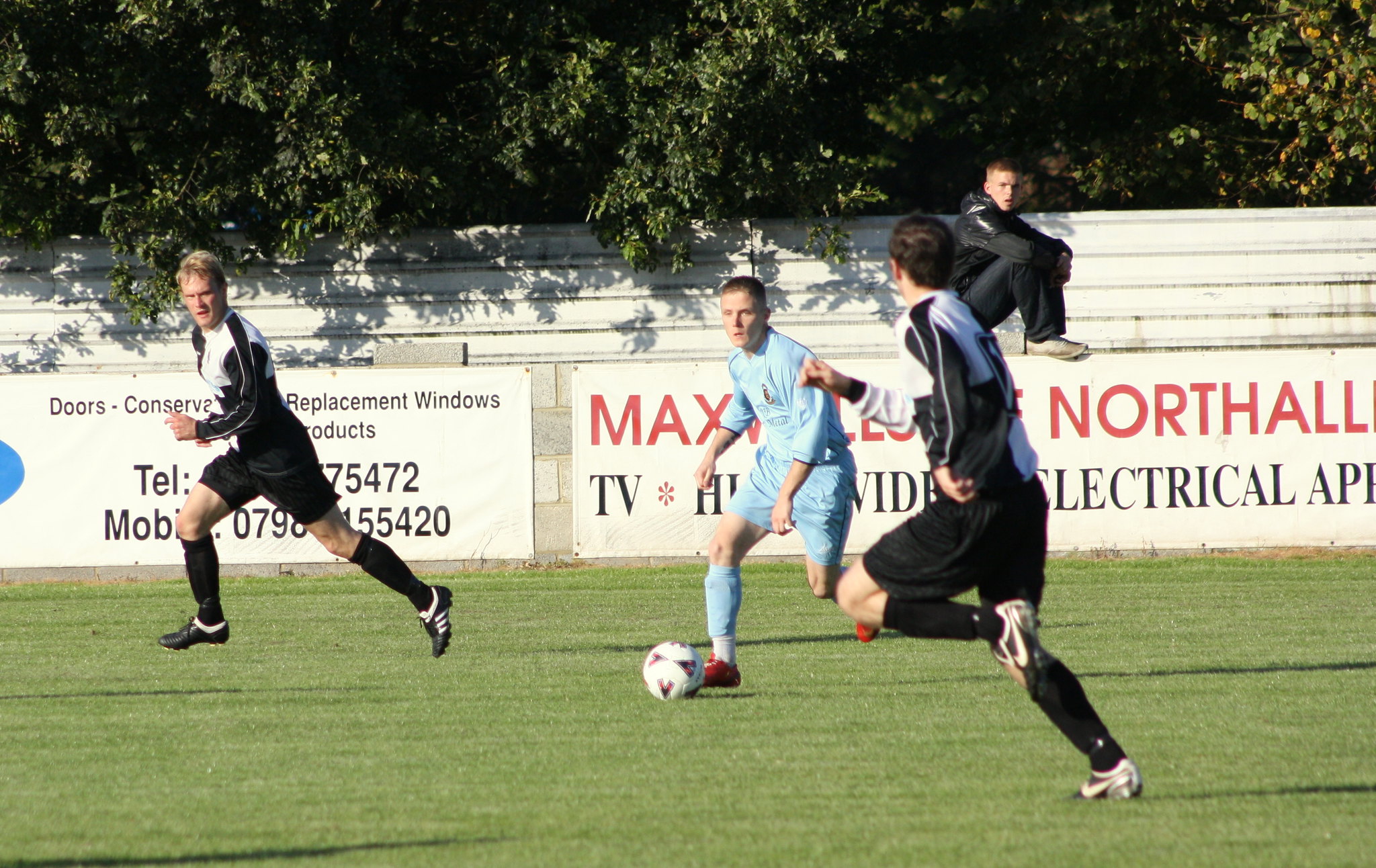In this detailed photograph set on a bright, sunny day, a high-paced soccer game unfolds on a well-maintained field surrounded by a distinctive large gray stone wall. Three young males are captured mid-run, converging towards a soccer ball, embodying the competitive spirit of the sport. The player on the left wears a sleek, black and white jersey, complemented by black shorts, socks, and black soccer cleats adorned with white stripes. In the center, a player in a full light blue uniform is poised to kick the ball, his movement accented by his striking red cleats. Another player in pursuit also sports a black and white uniform. Behind the field, a sparse audience seating area composed of multiple steps is visible, where a solitary spectator casually sits on the stone wall. This person, dressed in a black jacket and pants with dirty white shoes, faces towards the right, intently watching the game. The scene is further enriched by the backdrop of lush trees and various billboards advertising an assortment of products, hinting at a semi-professional or practice match. The energy and dynamics of the moment are palpable, showcasing the beauty and excitement of soccer.